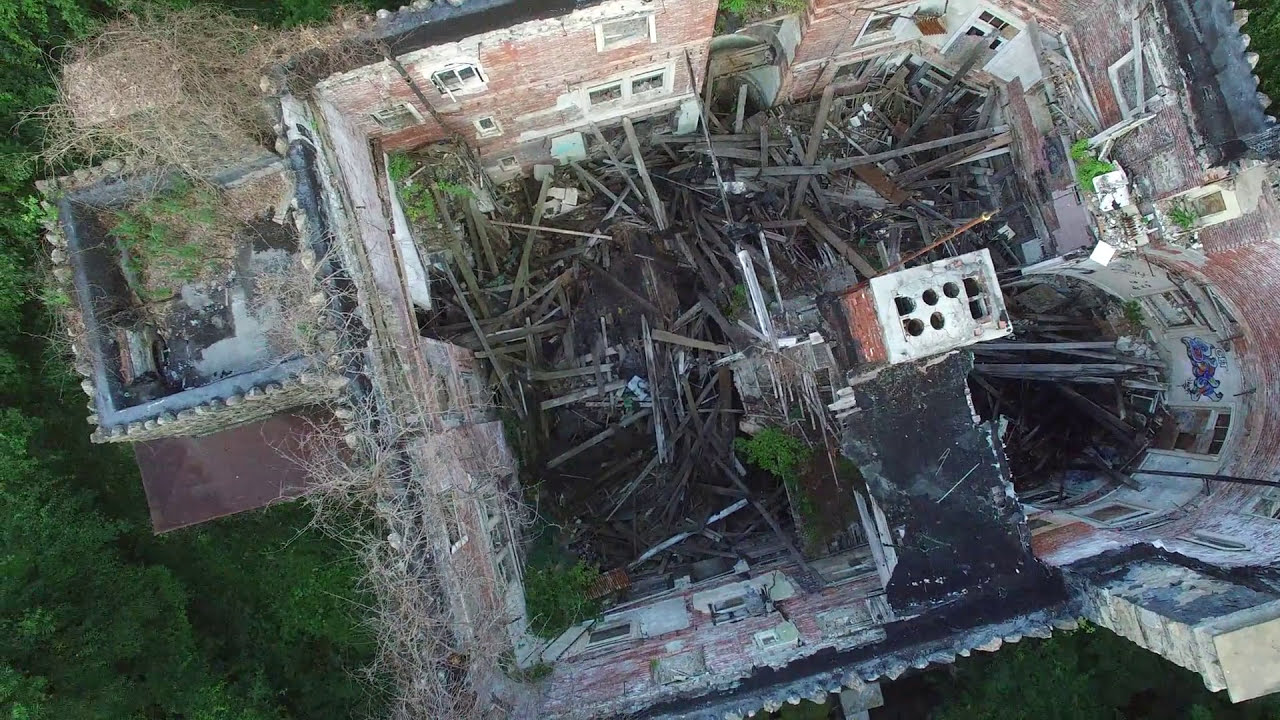The image captures an aerial, top-down view of a heavily damaged historic building, likely once a castle, constructed with red brick and stony rock walls. The exterior walls still stand tall, with visible remnants of at least three floors, including window sections on the upper levels. However, the roof has entirely collapsed, revealing the interior filled with large pieces of burnt timbers and lumber scattered around, suggesting a fire may have contributed to the destruction. The center of the building houses a partially intact chimney that stands amidst the debris, though it is punctuated with holes. The right side of the structure features a unique curved wall, indicating the presence of a spiral or regular tower in its original form. Adjacent to the main building, on the left, there is a smaller, square-shaped side building, positioned on slightly elevated ground. Unlike the main building, it lacks large timber debris, perhaps indicating only the removal of its roof. The main building's interior is now overgrown with dark, black soil and patches of grass, while the exterior surroundings are dotted with trees and other vegetation.